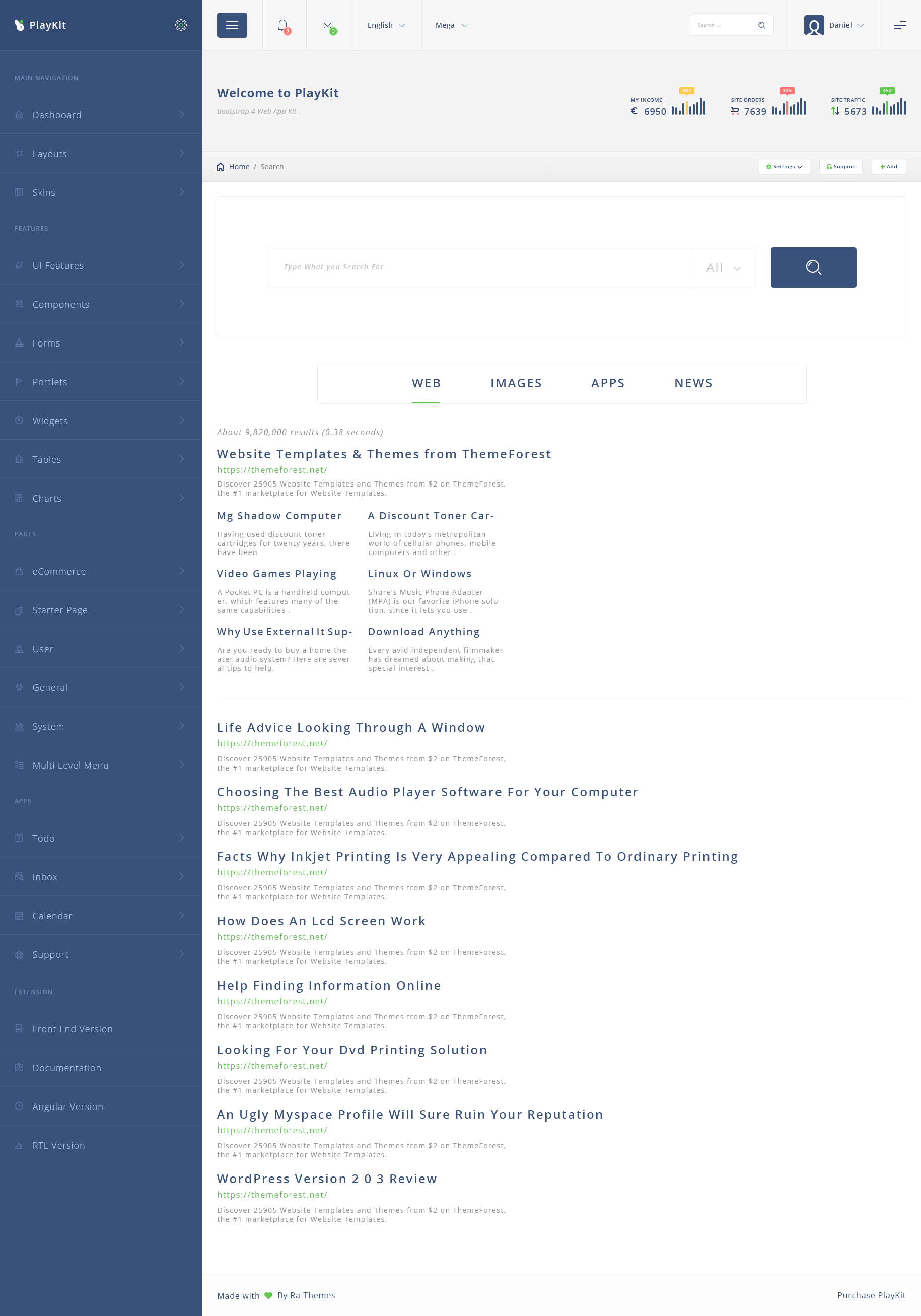This is a detailed and descriptive caption for the provided screenshot:

---

The screenshot captures a web page with a prominent blue sidebar on the left-hand side displaying a vertical menu labeled "PlayKit." The menu includes the following sections: Main Navigation Dashboard, Layouts, Skins, Features, UI Features, Components, Forms, Portlets, Widgets, Tables, Charts, Pages, E-Commerce, Starter Page, User, General, System, Multi-Level Menu, Apps, To-Do, Inbox, Calendar, Support, Extension, Front-End Version, Documentation, Angular Version, and RTL Version.

To the right of the blue sidebar, on a white background, the page header reads, "Welcome to PlayKit, Bootstrap and Web App Kit." Below this welcoming message, it presents three key metrics: "My Income: 6,950 Euros," "Site Orders: 7,639 Euros or 7,639 Orders," and "Site Traffic: 5,673." 

Further down, there are tabs for navigating different types of content: Web, Images, Apps, and News. The page also suggests various resources and topics from ThemeForest, such as Web Templates and Themes. Other highlighted topics include "MG Shadow Computer," "Video Games Playing," "YU's External IT Support," "Discount Toner Cartridges," "Linux or Windows," "Download Anything," "Life Advice Looking Through a Window," "Choosing the Best Audio Player Software for Your Computer," "Facts Why Inkjet Printing is Very Appealing Compared to Ordinary Printing," "How Does an LCD Screen Work," "Finding Information Online," "Look for Your DVD Printing Solution," "An Ugly MySpace Profile Will Sure Ruin Your Reputation," and a review titled "WordPress Version 2.0.3 Review."

---